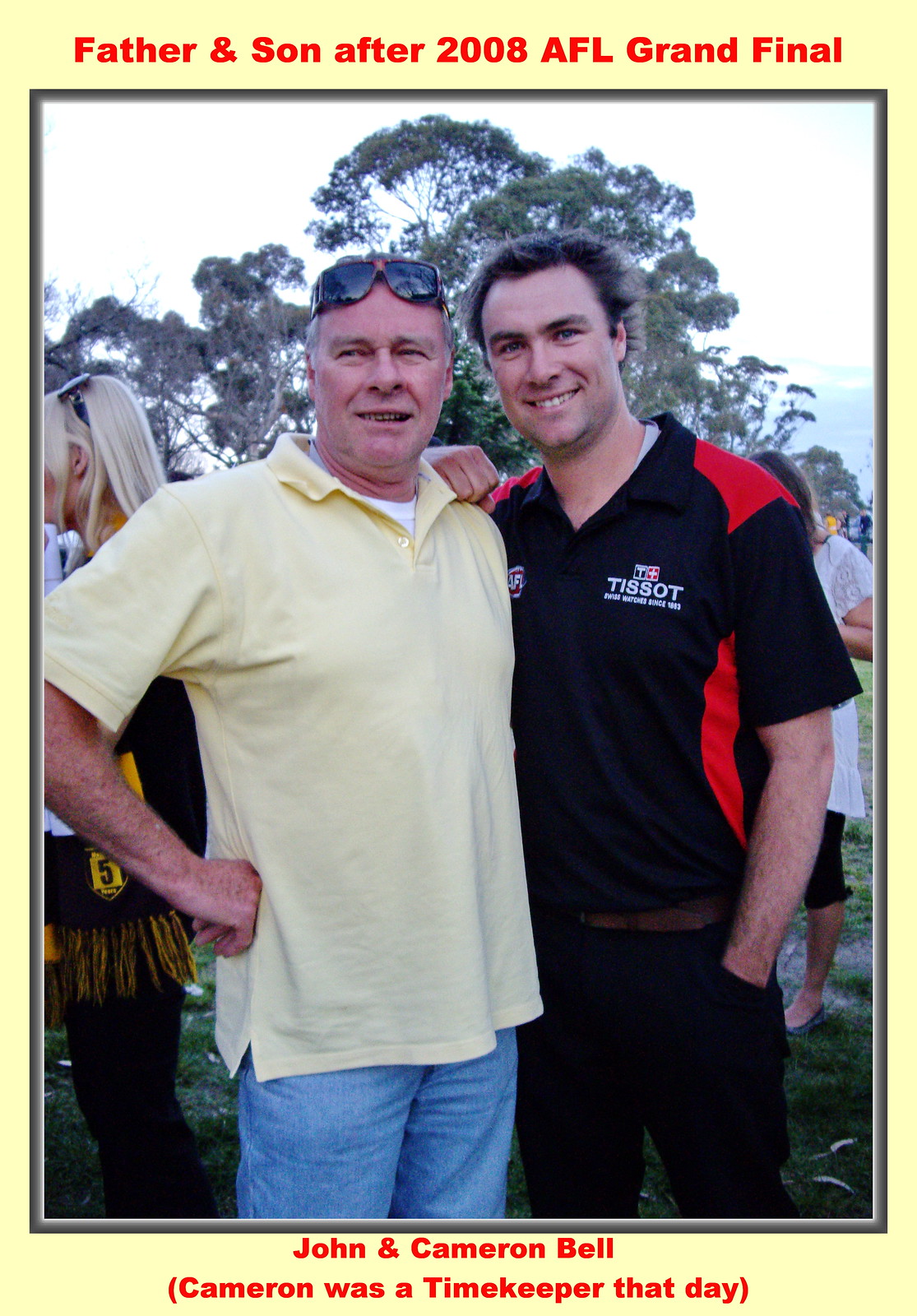This photograph captures a joyful moment between a father and son, John and Cameron Bell, taken after the 2008 AFL Grand Final. The photo, framed with a small black border and set against a yellow background, has inscriptions in red at the top and bottom. At the top, it reads "Father and Son after 2008 AFL Grand Final," and at the bottom, it names the subjects, "John and Cameron Bell," noting in parentheses that Cameron was a timekeeper that day.

In the forefront, John, the father, stands on the left wearing a yellow polo shirt over a white undershirt, blue jeans, and has sunglasses perched on his forehead. His right arm is resting on his hip, and he looks off to the left with a broad smile. Cameron, the son, stands to John's right, with his arm affectionately draped over his father's shoulder. He is dressed in a black t-shirt featuring red accents on the shoulders and sides, and the word "Tissot" emblazoned on the front. Cameron is also smiling, gazing directly at the camera, with one hand comfortably tucked into his pocket.

They stand on a grassy area, with a tall tree and a blue sky—or possibly a distant body of water—visible in the background. Behind John, a blonde woman with long hair wearing a black jacket with yellow tassels can be seen. The photograph exudes a sense of happiness and contentment, documenting a proud moment shared between father and son.